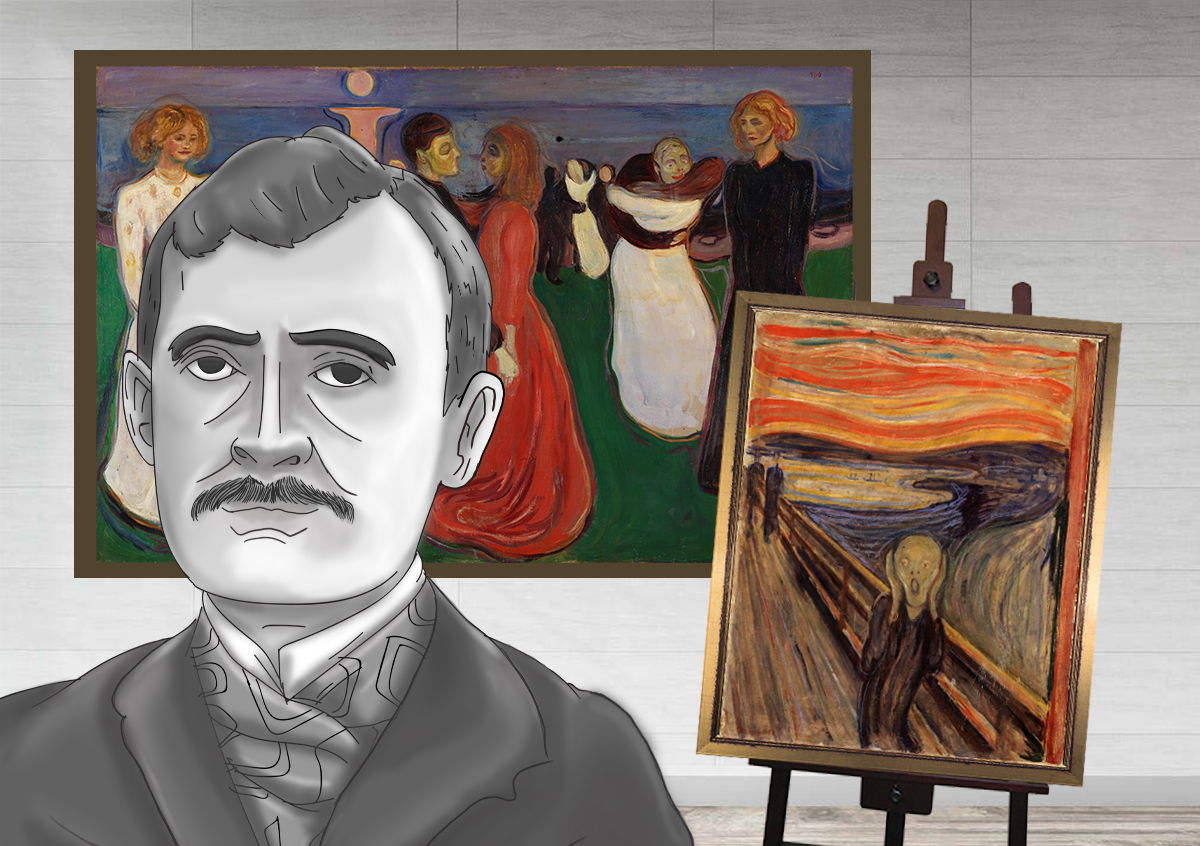In the foreground of this eclectic image composition, there stands a black-and-white illustration of a stern, mustached man dressed in old-fashioned attire, complete with a cravat and dark jacket. His cartoon-like line drawing is almost reminiscent of a historical figure, potentially the artist of the works displayed. Central to the scene is a vivid reproduction of Edvard Munch's renowned painting, "The Scream," propped on an easel. This piece vividly depicts a woman standing on a wooden deck over a river, her face contorted in horror, hands pressed to her cheeks, set against a dramatic sunset. Surrounding this striking centerpiece, the background showcases another artwork – a horizontal depiction of an outdoor gathering, with several women in long dresses, dancing and socializing, evocative of the styles from the 1800s. A red-orange clad woman, brown-haired, dances with a dark-haired man, while another woman in white and gold stands nearby. The simplistic, almost child-like execution of these artworks further adds to their intriguing allure, hinting at intentional artistic naivety possibly by the same artist, enhancing the gallery's display.